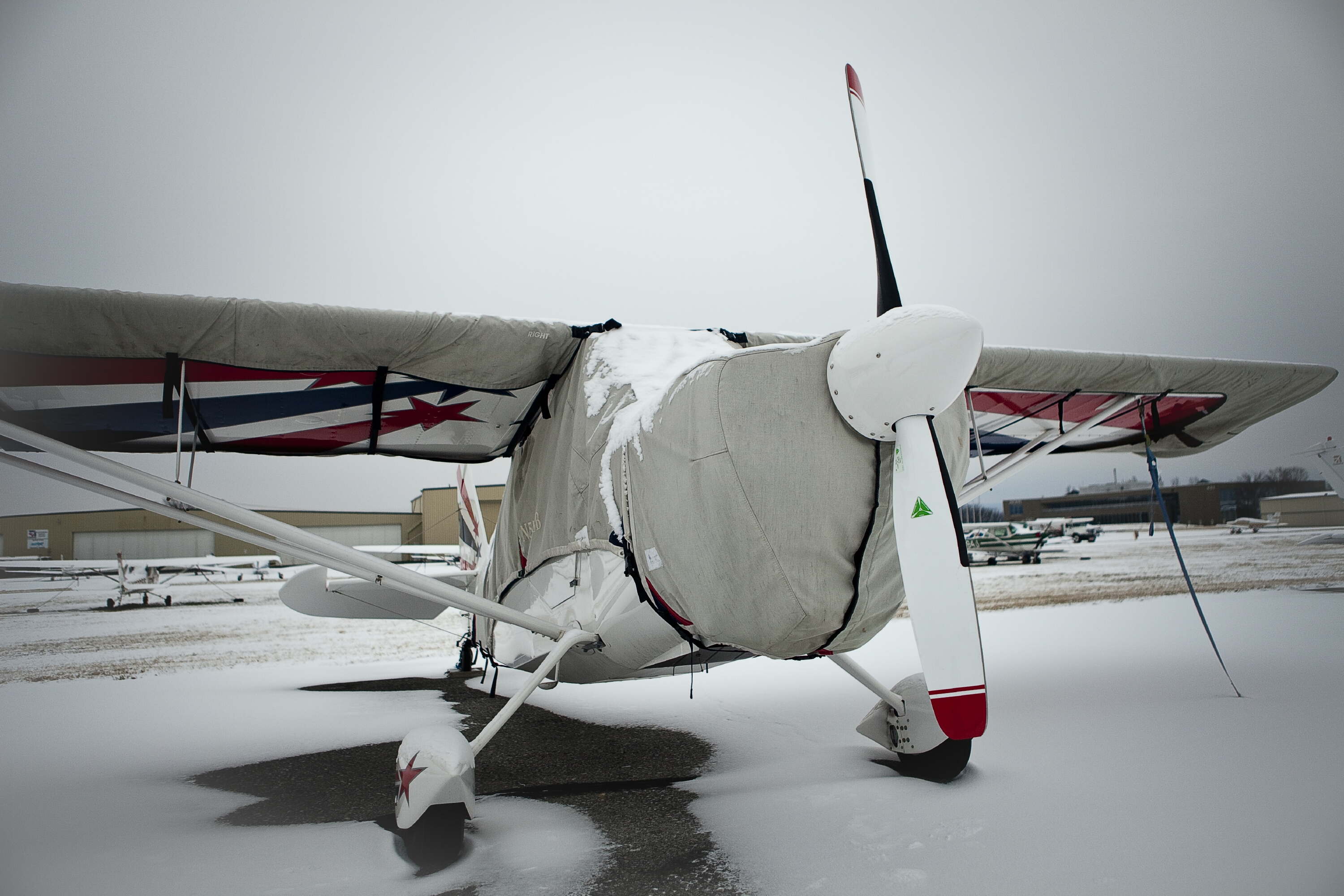The image captures a close-up view of a white propeller plane on a snow-covered tarmac, facing slightly to the right. The plane is wrapped in a grayish wooden canvas material covering its body, front nose, and windows, while parts of the wings are also wrapped but sections of the undersides remain visible. The wings sport alternating red and blue stripes, each terminating in stars matching the color of the stripes. Additionally, the tips of the lines on the wings each feature blue and red stars. The propeller, positioned towards the front right, has a distinctive coloring pattern with white at the base and red at the tips. Red and blue decorative lines and stars appear on the plane’s wings, as well as a prominent red star located on the landing gear housing. In the backdrop, there are several similar planes, and the sky appears overcast, adding to the wintry ambiance.